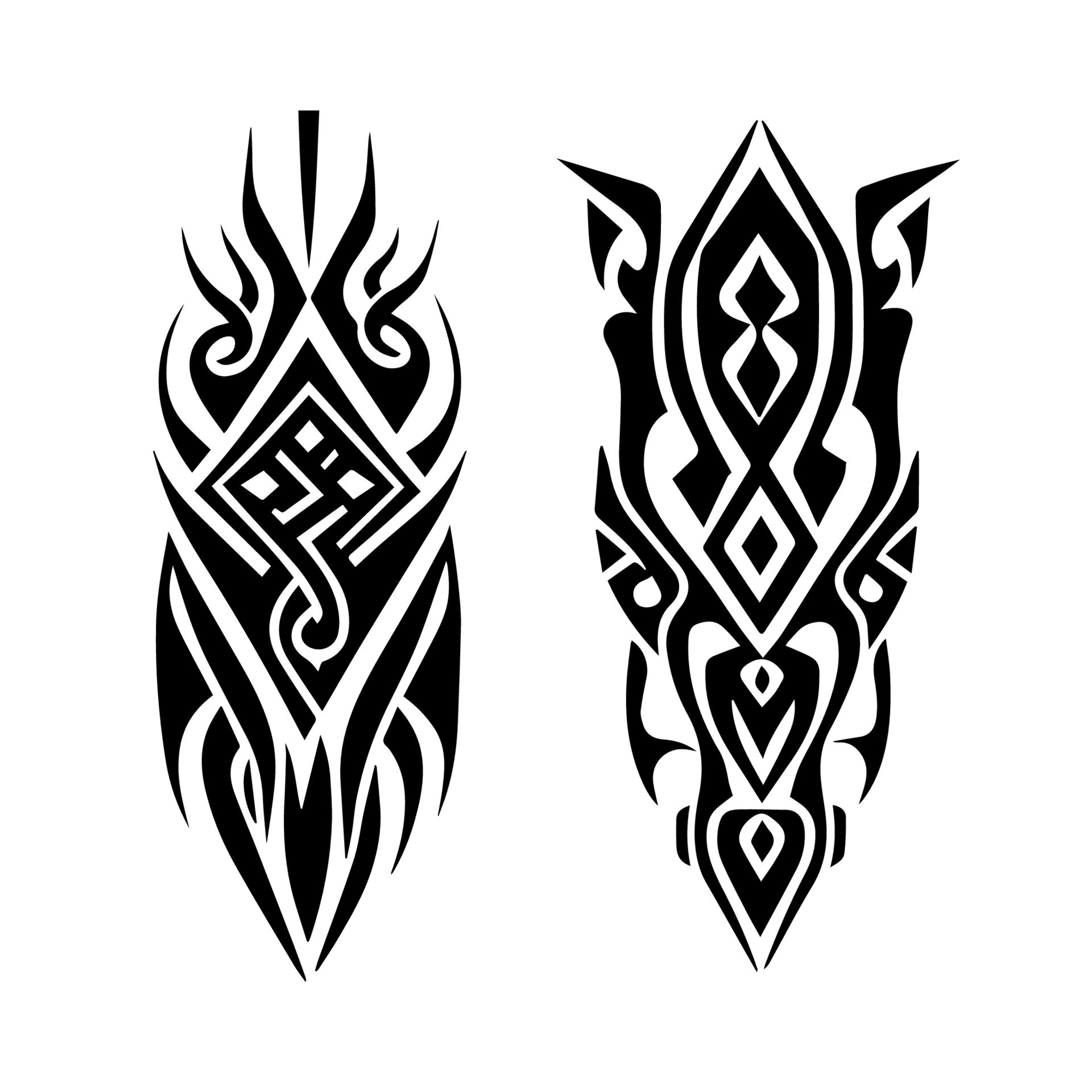The image showcases two vertically-oriented tribal designs set against a white background. Each design is approximately one and a half inches wide and four inches tall. They are predominantly black, with intricate patterns formed by the absence of white spaces, creating a stark contrast. Both designs feature a mix of curvy and angular elements, prominently displaying diamonds and swirls. The designs are reminiscent of tribal tattoos or masks and include stylized eyes and mouth regions. The left design has flame-like extensions at the top and a series of triangular and diamond shapes that give it a sharp, spiky appearance. The right design is more complex, with additional white patterns and prong-like extensions that curve down to meet a horn-like shape at the bottom, ending with a diamond at the tip. The tribal aesthetic is pronounced, with a strong emphasis on angularity and symmetry.